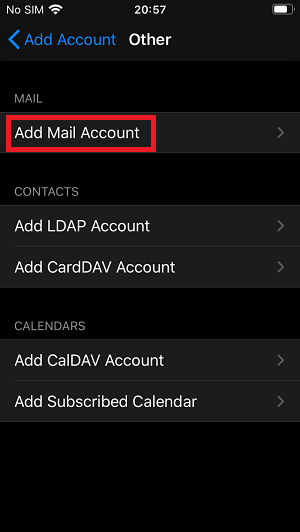Screenshot of a mobile device interface displaying a configuration screen. The top-left corner indicates "No SIM," and next to it, there are three bars of Wi-Fi signal strength. The time is shown as 20:57, and the battery icon suggests roughly 75% charge. The interface follows a dark theme with a predominantly black or gray background and white text.

At the top, in the middle, the category is labeled as "Other." Below it, a section titled "Mail" includes an option to "Add Mail Account," highlighted with a red rectangle (which appears to be a visual marker and not part of the actual UI).

Further down, under the "Contacts" section, there are options to "Add LDAP Account" and "Add CardDAV Account," each with dark gray backgrounds and right-facing arrows indicating further configuration options.

Finally, the "Calendars" section offers options to "Add CalDAV Account" and "Add Subscribed Calendar," similarly styled with dark gray backgrounds and right-facing arrows for additional settings.